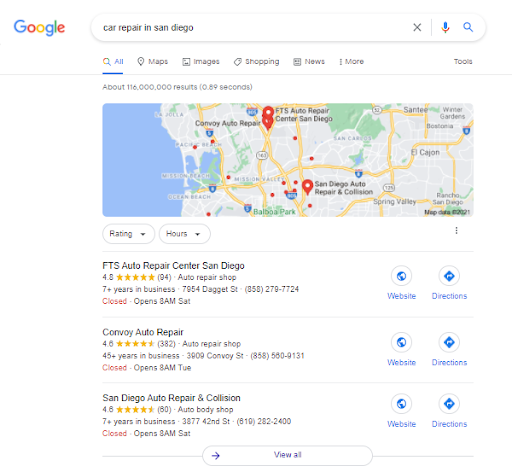The image displays a Google search results page featuring a query for "car repair in San Diego." The recognizable Google logo is prominently positioned at the top of the page, with the search term "car repair in San Diego" entered into the search field below. The "All" tab is highlighted in blue with an underline, indicating it's the active category, while other categories like "Maps," "Images," "Shopping," "News," and "More" appear in gray.

Just beneath the search bar, it states there are approximately 116 million results returned in 0.89 seconds. A map is visible, marking three locations with red pins, which correspond to three listings displayed below the map.

1. **FTS Auto Repair Center San Diego**
   - Rating: 4.8 stars from 94 reviews
   - Category: Auto repair shop 
   - Years in business: 7+ years
   - Address: 7954 Daggett Street
   - Contact: 858-279-7724
   - Status: Closed, opens 8 a.m. Saturday

2. **Convoy Auto Repair**
   - Rating: 4.6 stars from 382 reviews
   - Category: Auto repair shop
   - Years in business: 45+ years
   - Address: 3909 Convoy Street
   - Contact: 858-580-9131
   - Status: Closed, opens 8 a.m. Tuesday

3. **San Diego Auto Repair and Collision**
   - Rating: 4.6 stars from 80 reviews
   - Category: Auto body shop
   - Years in business: 7+ years
   - Address: 3877 42nd Street